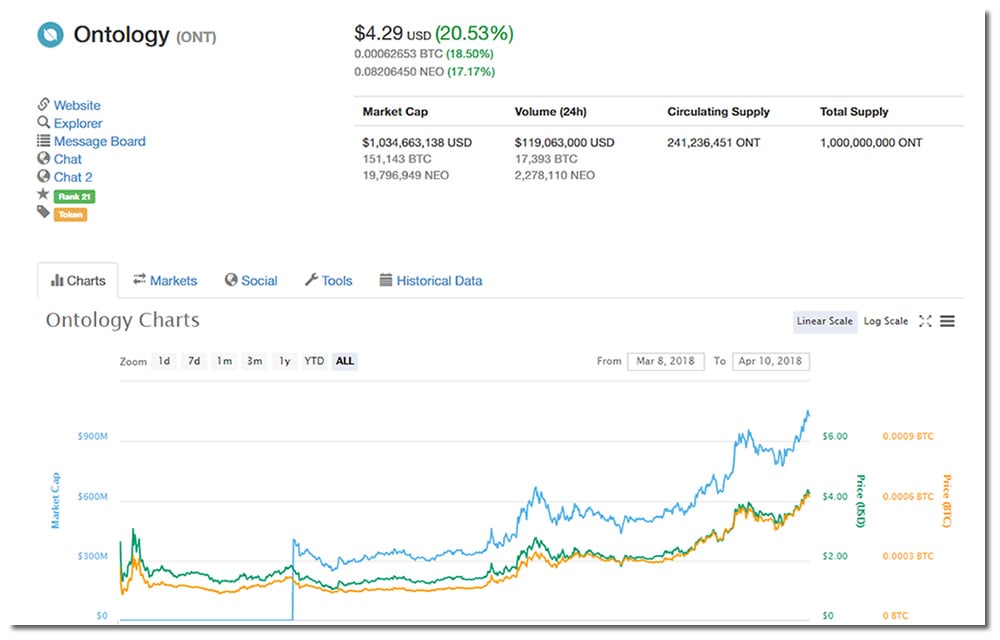**Detailed Caption:**

This is a computer screenshot with a white background. In the upper left-hand corner, there is a company logo. To the right of the logo, in bold black font, the word "Ontology" is displayed, and further to the right, enclosed in parentheses and in grey, is the ticker symbol "ONT." Positioned slightly left of the center of the screen is the current price, displayed as "$4.29" in bold black text. Directly below this price, the abbreviation "USD" appears in smaller, all-caps font, with a green percentage increase of "20.53%" in parentheses next to it.

Directly beneath this section, there are two rows showing small, detailed numbers for BTC and NEO, each accompanied by their respective percent changes in green. 

On the left side of the image, two lines below the price information, there is a vertical column of icons. Each icon is accompanied by a descriptive text in blue: "Website," "Explorer," "Message Board," "Chat," and "Chat 2." Adjacent to this column, there are two buttons: the first button is green with white text that reads "Rank 21," and the second button is orange with white text that reads "Taken."

Further down, a tab section is visible. The first tab, labeled "Charts," is grey, indicating it is the selected tab. The other tabs, namely "Market," "Social," "Tools," and "Historical Data," are in blue and have small icons to their left. Below these tabs, on the left side, it says "Ontology Charts" in grey. Dominating the lower portion of the screen is a detailed line graph featuring blue, green, yellow, and orange lines.